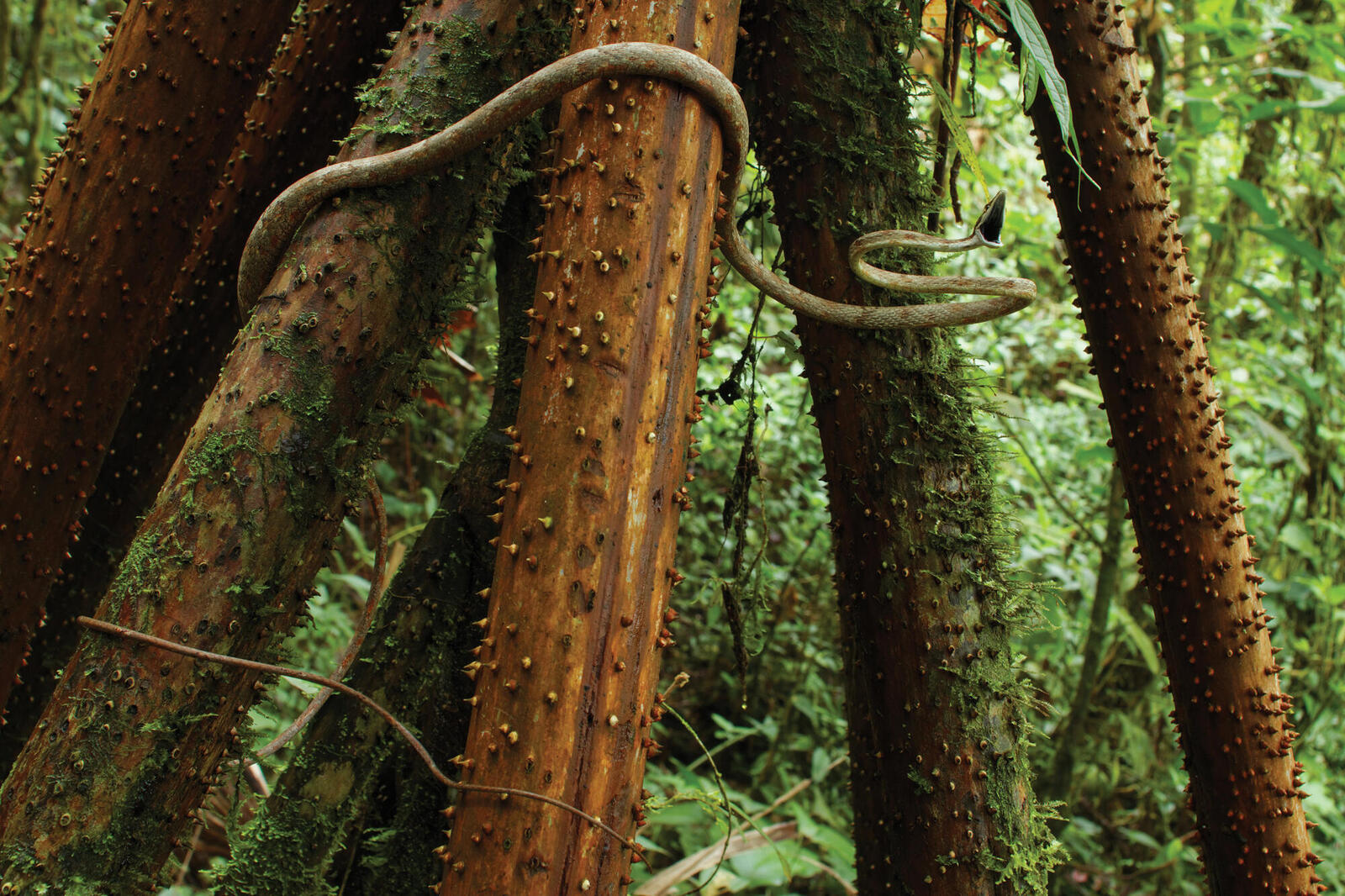The image depicts a dense jungle scene dominated by several thin, brown trees, some of which have small spikes and patches of green moss growing on their trunks. The focal point of the image is a large brown snake, approximately 4-5 feet long, with orange and red spots, wrapped around a couple of these trees. The snake has its mouth open, poised as if ready to strike, adding a sense of imminent action to the scene. The background is filled with lush green foliage, enhancing the dense, vibrant atmosphere of the rainforest setting. Scattered among the trees are various leaf-like objects and possibly branches or insects, contributing to the intricate and lively environment. The overall palette of the image features rich browns and greens, highlighting the natural beauty and complexity of the jungle.